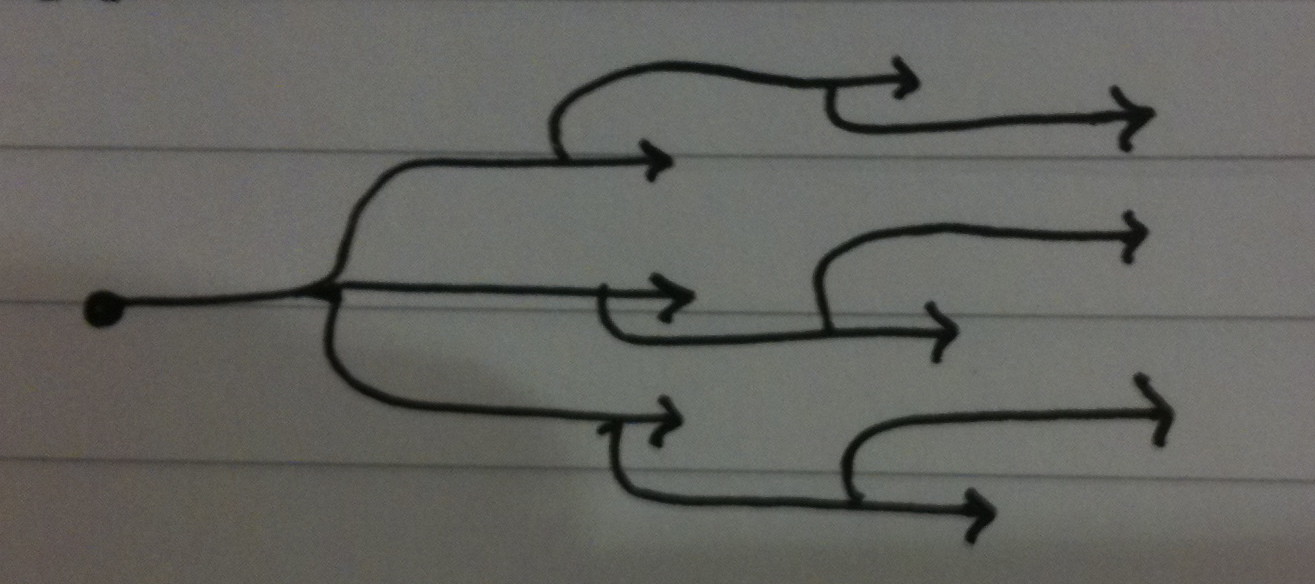This detailed drawing, depicted on standard white paper lined horizontally with three black lines, showcases a close-up view of intricate arrow designs. The paper's lined texture creates four white spaces, contributing to its organized appearance. The specific focus is on the center line, where, about an inch in, a prominent black circle anchors the composition. Extending from this circle, three smaller arrows radiate in a meticulous pattern.

The first arrow begins on the left, curving upwards to the right, forming a sharp arrowhead, then descending slightly before rising again to another point. It repeats this pattern once more, creating three distinct points.

The second arrow, positioned in the center, projects straight forward. It features a pointed tip, followed by a subtle leftward notch beneath it, continuing rightward to form another arrowhead. It consistently repeats this structure, ending with an upward deviation before its final arrow point.

The third arrow, starting at the bottom, descends and then shifts rightward to a point. Just before this arrowhead, it drops slightly, extends right, and forms another tip. It ultimately ascends again, concluding with an upward-right arrow point.

The delicate shadows cast by these arrows add a subtle depth, bringing the flat image to life with a refined touch.